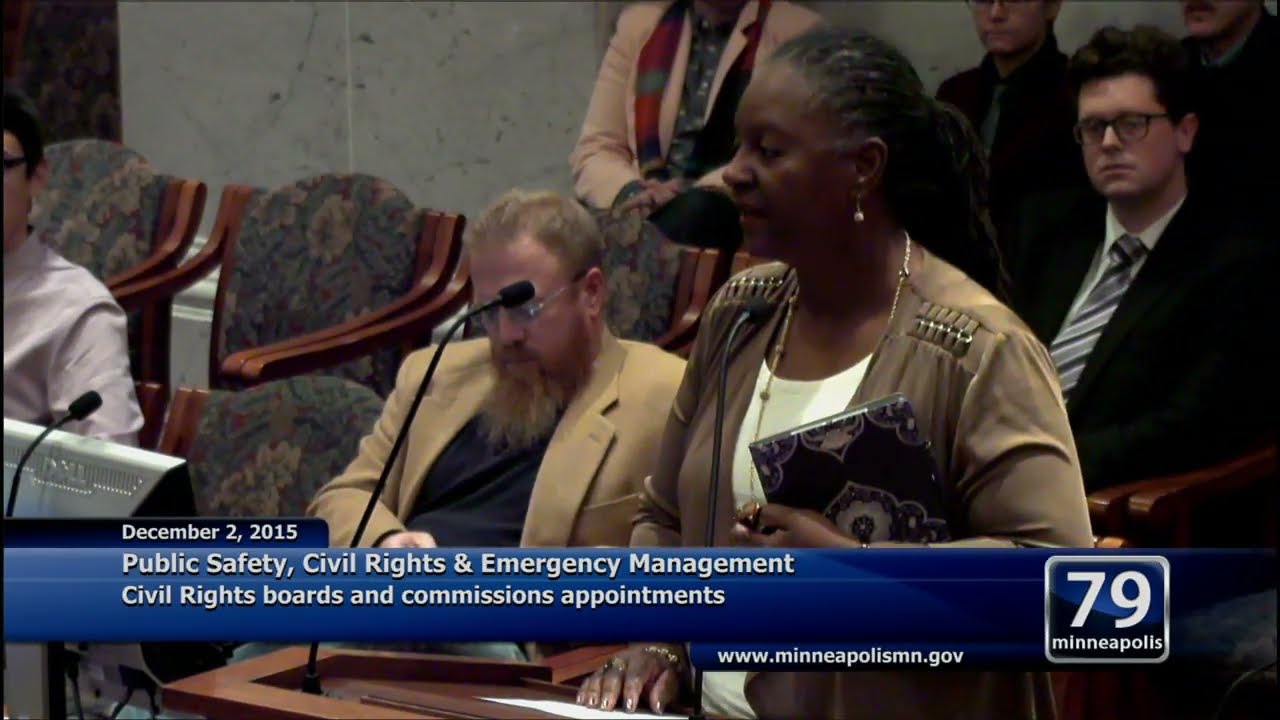The image is a screen grab from a news broadcast, dated December 2nd, 2015, as indicated by the blue text bar stretching across the bottom of the screen. The text mentions topics such as public safety, civil rights, emergency management, civil rights boards, and commission appointments, followed by the website www.minneapolismn.gov. In the lower right-hand corner, the number 79 and Minneapolis are enclosed in a square.

The main focus of the image is an African-American woman standing and speaking in what appears to be a courtroom or official meeting. She has black hair tied back into a ponytail and wears a white collared shirt under a light tan long-sleeve jacket. She appears serious and is adorned with gold earrings and a gold necklace. In her left arm, she clutches a patterned notebook close to her chest, while her right hand rests on a piece of white paper on top of a dark brown podium. She speaks into a thin black microphone.

Behind her, several individuals are seated and watching. Directly behind her, a man in a black suit, white shirt, and tie sits attentively. To the left, a man with blonde hair and a beard, dressed in a beige blazer over a black shirt, sits near a row of unoccupied floral-patterned chairs. Another man, partially visible and wearing a white shirt, sits farther to the left, looking at the speaking woman. The room has a mixture of filled and empty chairs, with a visible computer screen in front of one of the seated individuals.